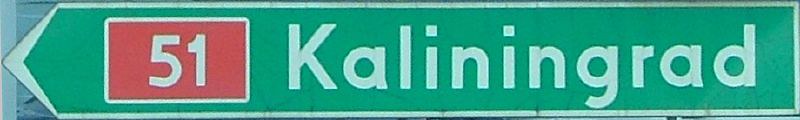The image depicts an exceptionally wide road sign, approximately six times wider than it is tall, set against a green background characteristic of road signs. The large, off-white arrow in the center points left, directing towards Kaliningrad, which is prominently written in bold white lettering. Positioned to the left of the arrow, there is a number "51" on a medium red rectangle, itself bordered by a white outline, further accentuated by an additional white box around the red rectangle. The sign is framed with silver detailing along its edges but contains no other significant text or imagery.